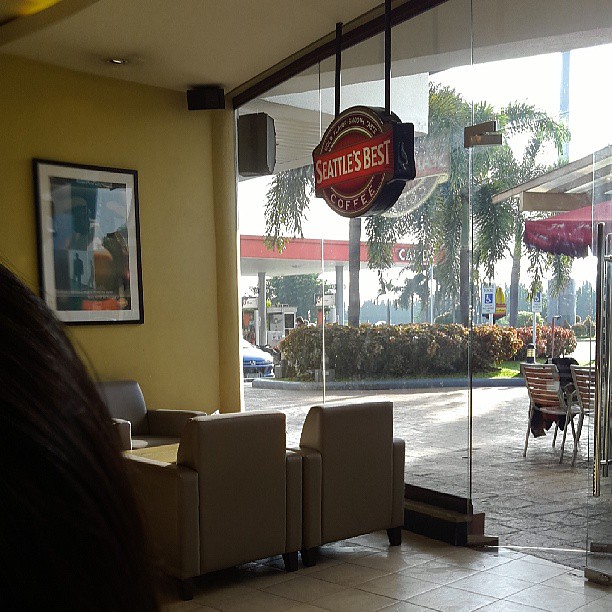The photograph captures a cozy cafe scene, viewed from inside a coffee shop marked by a large sign proclaiming "Seattle's Best Coffee." The cafe is adorned with cushioned seats and features a yellow wall to the left with a hanging movie poster. Through the mostly glass wall, we see a small patio with empty tables, chairs, and an umbrella on the right side of the frame. A cobblestone walkway leads to a red gas station visible in the distance. A maroon overhang provides shade for the patio area. Inside, a person is seated to the left, and another person's black hair is visible in the bottom left corner, suggesting they are close to the photographer. Outside, someone is seated, and another figure is standing nearby, though their features are not clear. The door to the cafe is slightly open, and it appears to be a sunny day with a light overcast. The overall atmosphere suggests a welcoming and relaxed environment where one can pause for a cup of coffee.